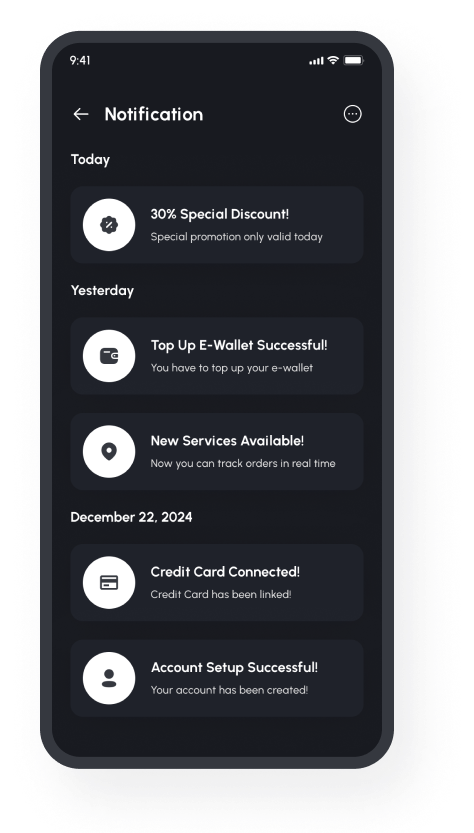This image is a layered screenshot of a cell phone display, likely from an advertisement, captured multiple times. One can discern the distinct rim of the phone, indicating a meta-screenshot effect. The top of the screen shows it's 9:41 with full bars of service and Wi-Fi, and a battery at 100%.

Prominent on the screen is a back arrow and the bold white text "Notification". Below is a series of notifications in white circles. 

1. The first circle features a black badge with a "Z" inside on a white background. It reads "30% off special discount!" followed by "Special promotion only valid today."

2. The second notification has a wallet icon and states "Top up e-wallet successful" and "Top up your e-wallet".

3. The third circle has a black location tag and reads "New services available! Now you can track orders in real-time."

4. The fourth notification, dated December 22nd, 2024, with a credit card icon, announces "Credit card connected. Credit card has been linked."

5. The final circle, with a person icon, states "Account set up successful. Your account has been created."

The display uses dark mode, with all fonts in white against a black background, enhancing visibility and contrast.